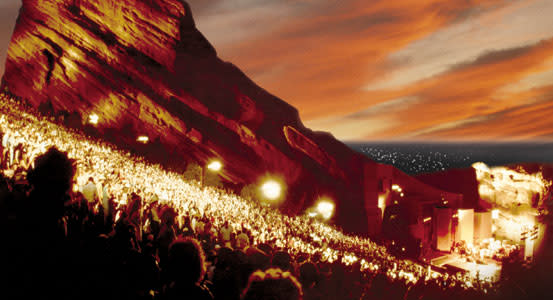The image depicts what appears to be an outdoor concert at the iconic Red Rocks Amphitheatre in Colorado, captured either in a photograph or as a painting. The scene is viewed from above, showcasing a sloped audience area filled with countless concertgoers, some of whom are holding up lights—possibly flashlights, cell phones, or candle lighters. The well-lit stage is situated at the bottom right, equipped with a screen and set against a dramatic, irregularly-shaped natural stone wall that rises higher toward the top of the slope. The rocky terrain is rugged and uneven, reflecting the light from the audience. Beyond the stage, the backdrop reveals a stunning sunset sky, transitioning from pale blue to bright orange with hints of purple amidst the clouds. The overall ambiance is highlighted by the interplay of light against the natural features, creating a picturesque and vibrant evening scene.